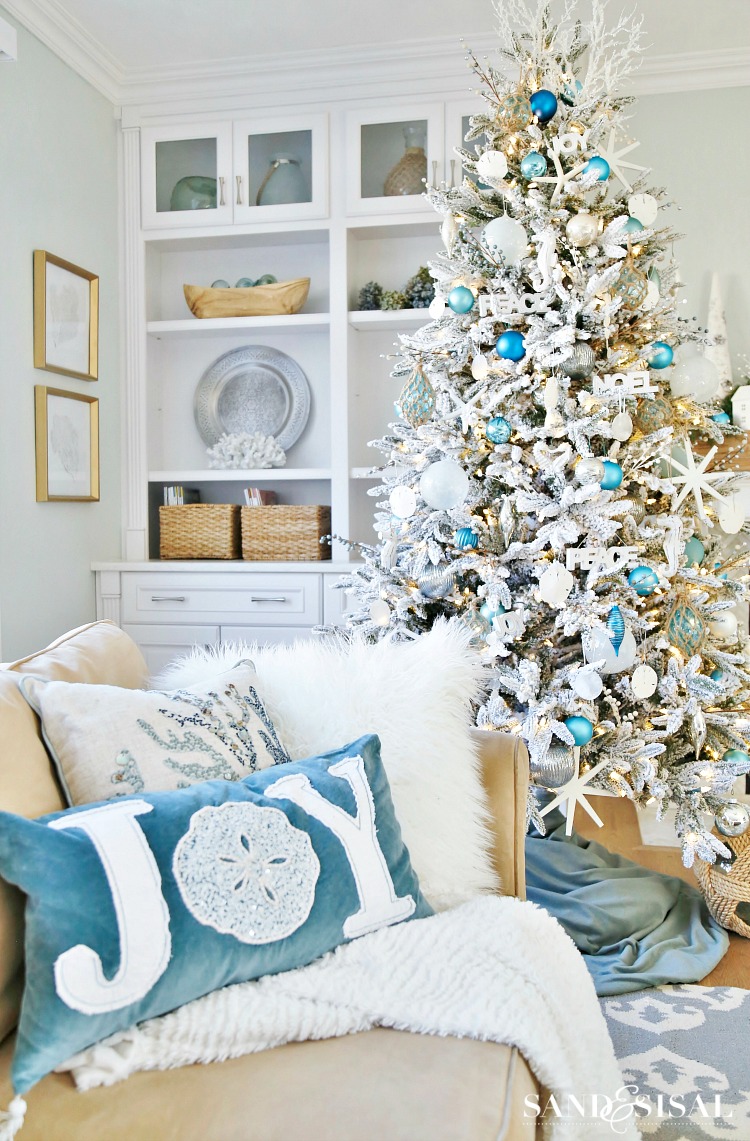The image depicts a festive and modern Christmas scene in a home, specifically a living room. The walls are painted a bright blue, complemented by a white ceiling and built-in white cabinetry with silver-handled drawers. The cabinets feature clear glass openings showcasing baskets, urns, and decorative plates, while gold-framed pictures adorn the wall to the left. Central to the image is a tan couch accented with a furry white throw, a white furry pillow, and a silvery branch pillow partially obscured by a rectangular pillow that prominently displays the word "Joy" in white letters, where the "O" is designed to resemble a scalloped doily.

To the right, a tall Christmas tree dominates the scene, its frosted white branches adorned with blue decorations, icicles, and numerous ornaments, creating a white and light blue color theme. A cold frosty blue throw lies beneath the tree, resting on a neutral brown rug that extends into a blue and white patterned rug below the sofa. Overall, the image captures a celebratory and festive ambiance typical of the Christmas holiday, characterized by cozy and elegant decor.